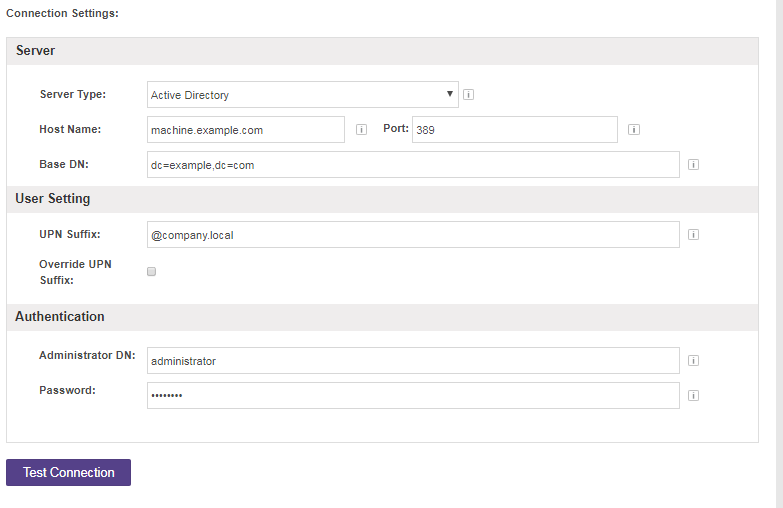The image depicts a configuration panel for server connections. In the upper-left corner, the title "Connections" is displayed. Below it, on a gray band, the word "Server" is written in black font. Underneath, on a white background, the label "Server Type" is followed by a drop-down menu showing "Active Directory." 

Next, the label "Hostname" is visible, accompanied by the text "machine.example.com" in the corresponding data field. To the right, a field marked "Port" contains the number "389." Below, the label "Base DN" is displayed, and the data field reads "DN=example, DC=com."

A gray stripe marks the next section, labeled "User Settings" in black. On a white background, the caption "UPN Suffix" is followed by the text "@company.local" within its data field. An option to override the UPN suffix is available, indicated by an unchecked gray box next to "Override UPN Suffix."

Following this, another gray strip appears with the label "Authentication" on the left. Beneath this, on a white background, the label "Administrator DN" is displayed, with "administrator" in the respective data field. Below that, the label "Password" is next to a concealed password field. At the bottom left, a blue button labeled "Test Connection" with white font can be seen.